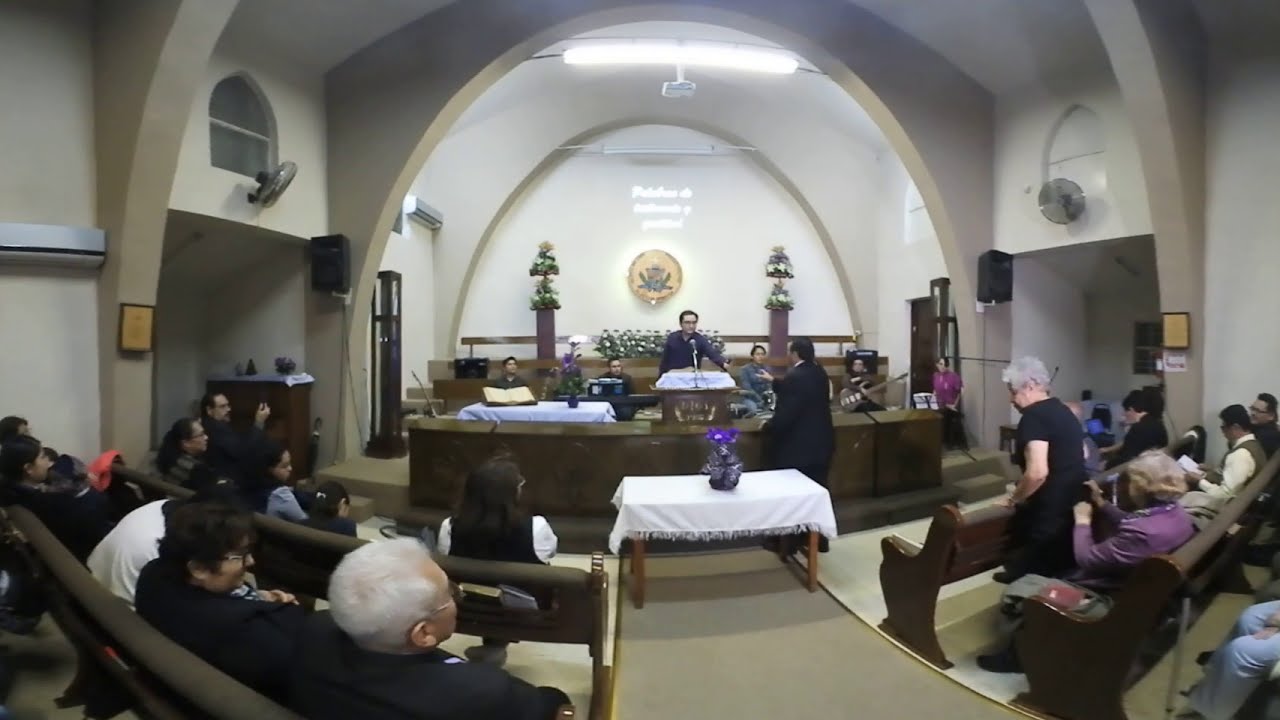The photograph captures the interior of a church, likely situated in a warm country such as in South America. Taken from the perspective of the third pew, the image features beige walls, tan arched ceilings, and a slight fish-eye effect emphasizing the curvature of the space. The congregation, mostly composed of elderly individuals with gray hair, fills the wooden pews on both sides of the aisle leading up to the main area.

At the forefront, a pastor or priest stands at a podium on a raised wooden platform, speaking into a microphone. The stage area includes a table adorned with a white tablecloth and a black vase containing purple flowers. Surrounding the speaker are several steps and additional people, including four individuals seated and another man in a suit conversing with the speaker.

The church is equipped with various fixtures: black fans attached to the walls for cooling, speakers for sound amplification, and a white fluorescent light illuminating the speaking area. Musical accompaniment is provided by musicians, with one visible holding a guitar in the background. The overall scene suggests a lively, well-attended service, possibly a baptism.